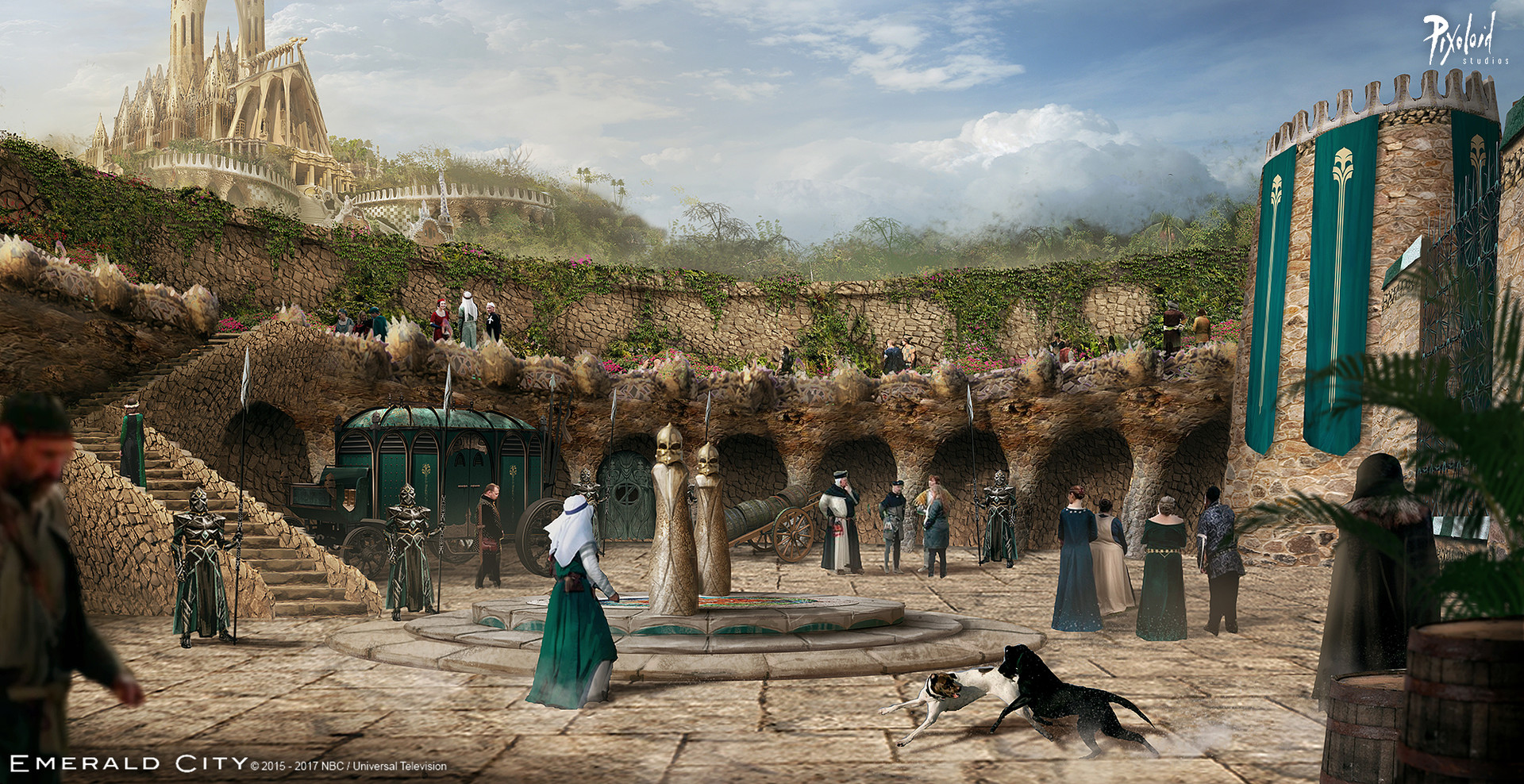The image depicts an intricate painting set in the medieval era, showcasing a vibrant town square. At the center of the square, there's a prominent fountain adorned with two statues of helmeted soldiers, around which approximately 20 people are gathered, dressed in period-appropriate medieval clothing. The background reveals armed guards in full armor, armed with spears, and a chariot. The scene is framed by castle walls and towers, with a distant view of what seems to be a church or more castle structures. A blue sky with scattered white clouds, particularly concentrated on the left, adds to the overall atmosphere. The painting also includes two playful dogs in the foreground. A signature, possibly “pixeloid,” is noted at the top, near an abstractly depicted castle built into a mountain. The ground is a mix of concrete and squares, indicative of a bustling courtyard, with medieval head coverings and Roman-inspired elements. The environment evokes a blend of King Arthur and Game of Thrones settings, rich with historical and fantasy vibes, aptly named "Emerald City."